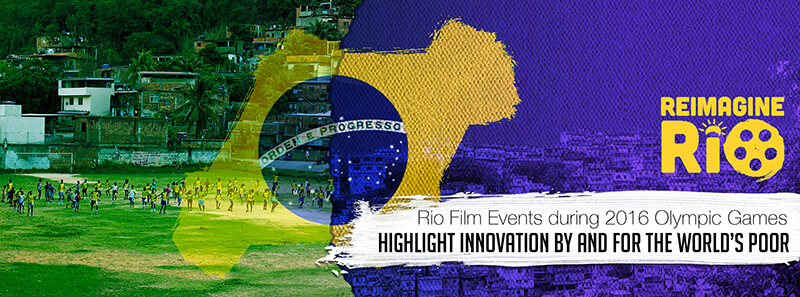This rectangular advertisement poster, titled "Reimagine Rio," prominently features a harmonious blend of deep purple and yellow hues on its right side, symbolizing innovation amidst the favelas of Brazil. The text "Reimagine Rio" is strikingly displayed in yellow with a film reel cleverly incorporated into the letter 'O'. Below it, a white banner states, "Rio film events during 2016 Olympic Games highlight innovation by and for the world's poor." Further details reveal the Brazilian flag elements subtly integrated over the purple overlay, featuring the yellow diamond, blue globe, and the inscription "Ordem e Progresso" with stars. On the left side, the image portrays children in a grassy field, likely playing soccer, clad in vibrant yellow and other colors. The background reveals Latin American housing structures, typical of Rio's favelas, marked by various elevations. This juxtaposition of artistic elements and real-life imagery captures the essence of cultural events occurring during a time of global unity and celebration.